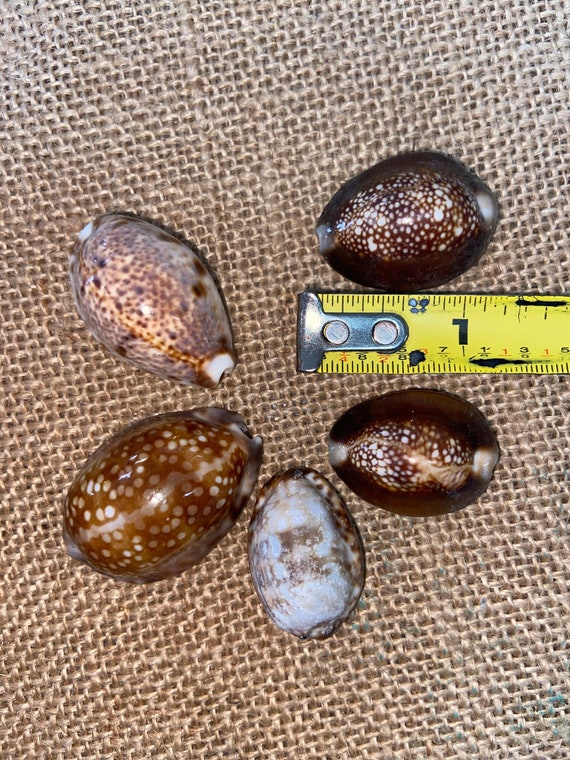The image depicts five oval-shaped seashells arranged on a rough brown fabric surface, likely resembling canvas or netting. Each shell displays unique colors and patterns: one has light brown speckles on a white background, another has white speckles on a brown background, and a third has a rough texture, possibly worn down by exposure to waves and water. The last two shells feature a distinctive brown ring with a pattern of brown and white speckles inside. To the right-hand side of the frame, a yellow tape measure is visible, indicating that the seashells are approximately one inch in length, providing a sense of scale.